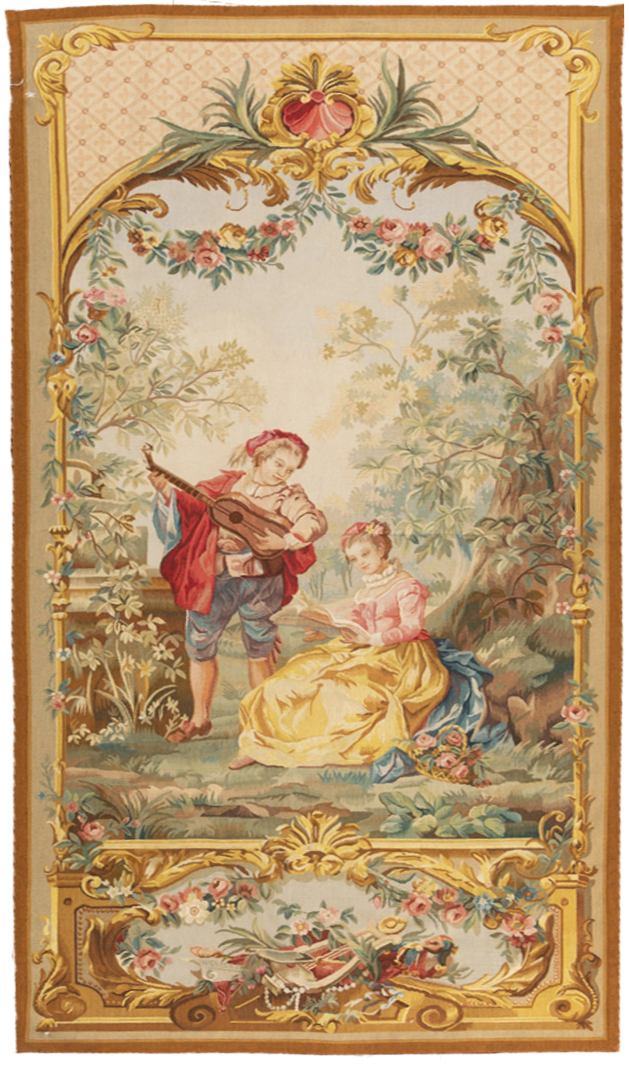The image appears to be a detailed tapestry rendered in a pale, painterly style, predominantly in tan, gold, and brown hues, with a touch of vibrant colors. At its center, there is a depiction of a serene forest scene. A woman, dressed in ornate old-fashioned clothing—a large, gold skirt and a high-necked, long-sleeved pale pink top—sits at the base of a tree, absorbed in reading a book. Beside her stands a man clad in short pants and a distinctive red cloak, playing a lute-like instrument. The scene is rich with nature, surrounded by trees and foliage, with an abundance of flowers adding a whimsical touch. The tapestry is encased in an ornate gold and beige border, further adorned with intricate patterns and floral motifs.